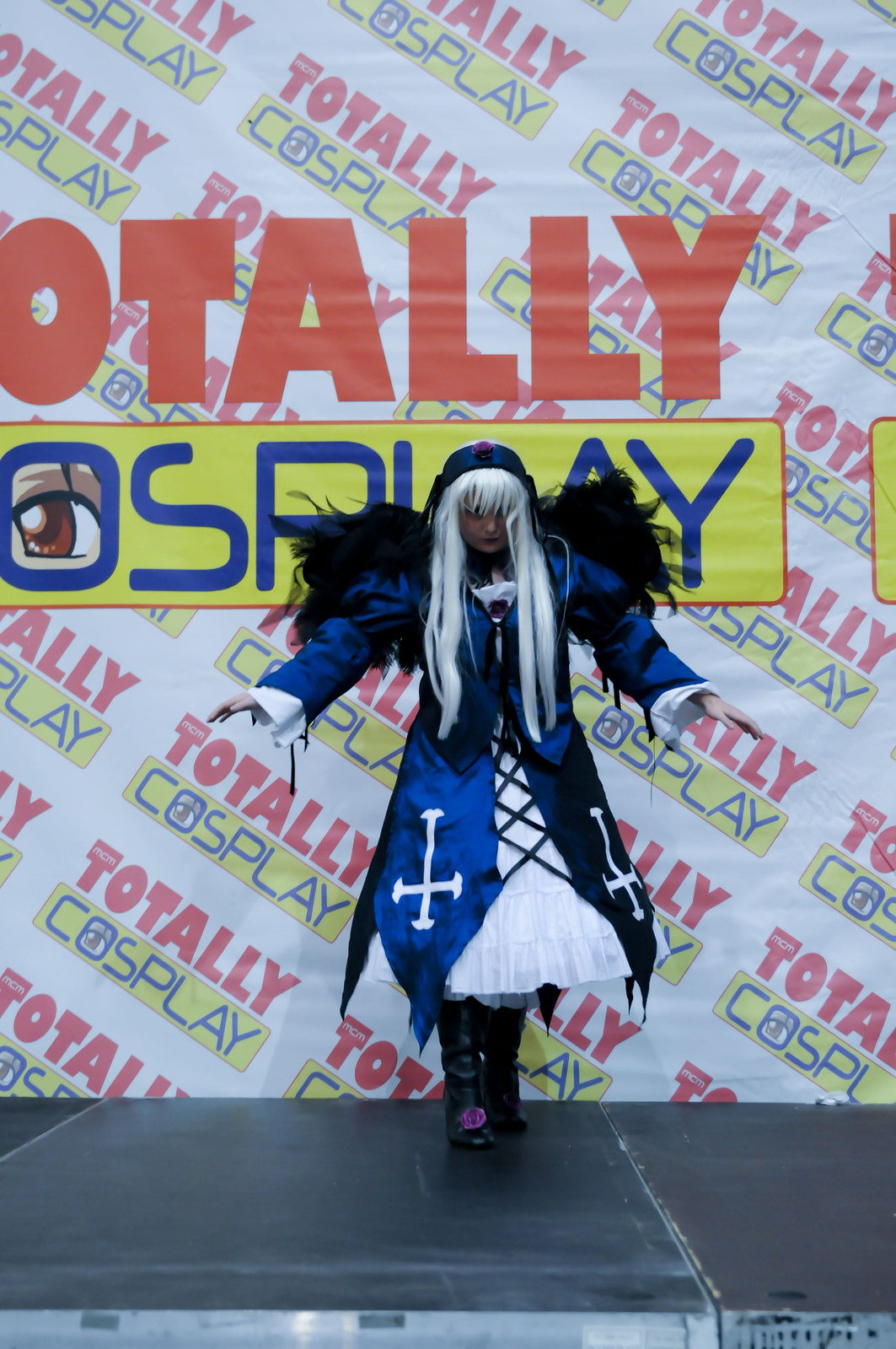The image features a cosplay performer standing on a gray stage, dressed in an incredibly detailed and exotic outfit. She wears a stunning long silver-gray wig with bangs and flowing strands framing her face. Her ensemble includes a striking long silver and white dress with a dark blue silk or satin coat cape that has black trim and crisscross lacing across the front. The coat cape also features long sleeves that reveal a white garment underneath, ending in a handkerchief hem. Notably, the base of her skirt showcases large inverted white crucifixes. Complementing her look, she sports elevated black boots that reach just below the knee, one of which has a red detail on the top.

Adding to the ethereal quality of her appearance, the performer has black feathery wings attached to her back. She is depicted in a dynamic pose with her hands outstretched. In the background, there is a large wall with a repeating angled graphic that reads "TOTALLY COSPLAY" in alternating red and blue letters against a yellow backdrop. The cohesion and intricacy of her outfit make her a standout figure in the scene.